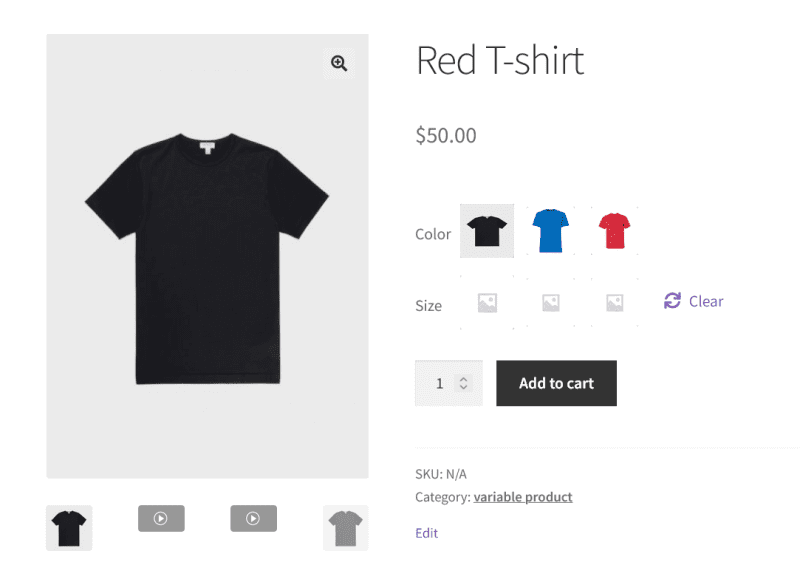The image showcases an online shopping interface for a black t-shirt prominently displayed on the left side. In the top right corner, a small magnifying glass allows users to zoom in on the t-shirt. Below this, various navigation buttons enable users to view alternate angles or versions of the t-shirt.

On the right side of the interface, the text mistakenly labels the product as a red t-shirt, even though the image displays a black one. Underneath this mislabel, the price is listed as $50. Below the price, there are three thumbnail images displaying the t-shirt in different colors: black, blue, and red. 

Further down, there is a size selector featuring three icons indicating the available sizes. Adjacent to the size options, a clear button allows users to reset their selections. Below this section, a quantity selector with up and down arrows lets users choose the number of t-shirts they wish to purchase, with the default quantity set at one.

Finally, a gray button with white text labeled "Add to Cart" enables users to complete their selection process by adding the chosen t-shirt, in the specified color, size, and quantity, to their shopping cart.